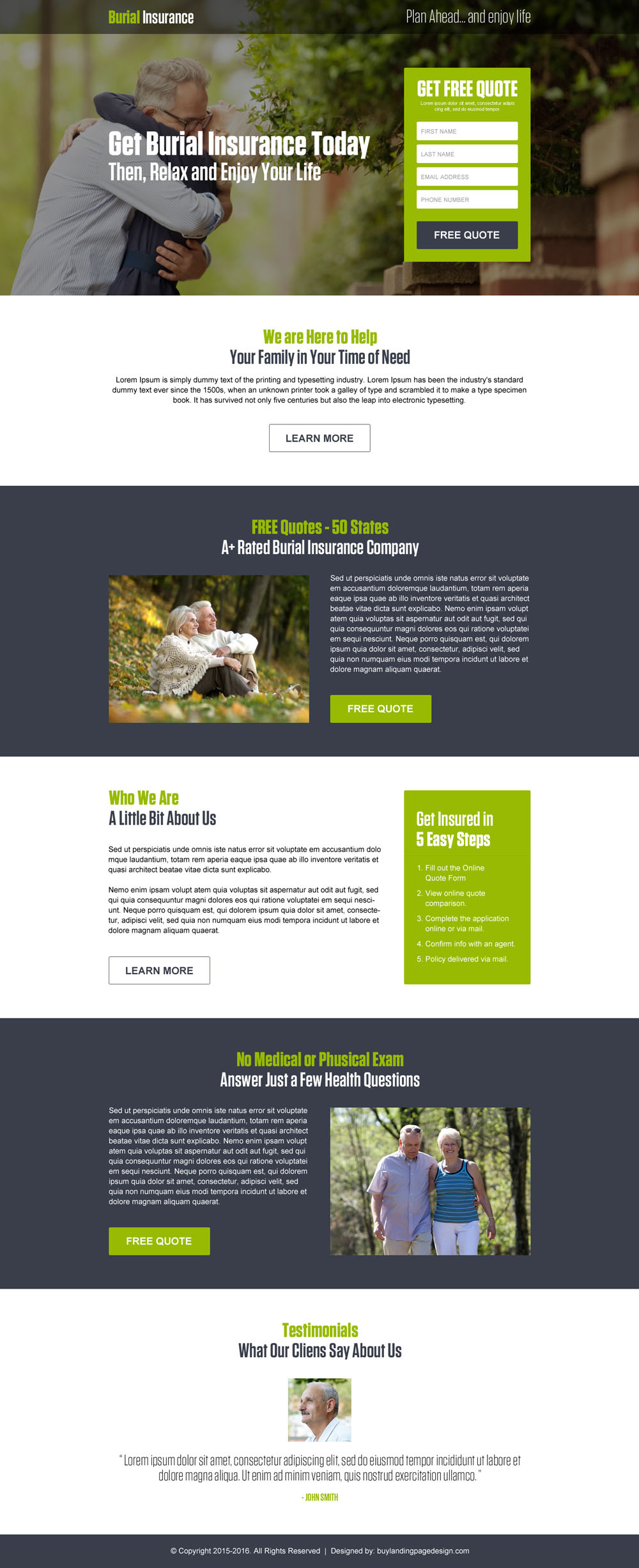The webpage for burial insurance features a series of four images, each accompanied by text, providing a detailed understanding of the service being offered. At the top of the page, there is a rectangular section with bold text declaring, "Get Burial Insurance Today." Below this, a comforting tagline reads, "Calm or Relax and Enjoy Your Life." The image in this section showcases an elderly couple with gray hair hugging each other warmly. The elderly man, dressed in a long-sleeve shirt and glasses, is more prominently visible than the woman. On the right side of this image, a call-to-action urges visitors to "Get Free Quotes," prompting them to enter their first name, last name, email address, and phone number to receive a free quote.

Beneath this main image, an informative text reassures visitors, stating, "We are here to help your family in your time of need," alongside some additional words that are somewhat difficult to read. This text is followed by a reiteration, "More and More."

The second image features the same elderly couple, now seated on a grassy area adorned with autumn leaves. The accompanying text promotes the burial insurance service with the words, "Free Quotes - 50 States, A+ Rated Burial Insurance Company."